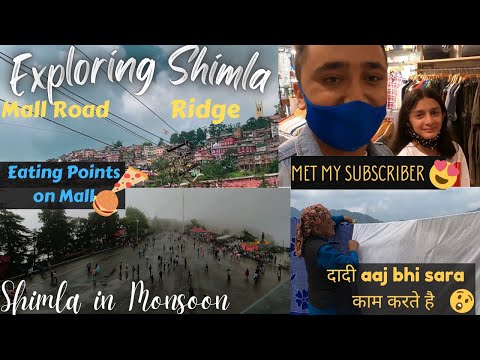This image appears to be a social media collage from an influencer, bordered by black at the top and bottom. The collage consists of four distinct photos. The upper left photo features a hillside view with greenery and numerous red brick houses, captioned "Exploring Shimla" in white text and "Mall Road Ridge" in yellow. The upper right photo depicts a man in a light blue shirt and blue COVID mask, standing in a store with a woman with long brown hair behind him. This image is labeled with "Met My Subscriber" in a black box with yellow text and a heart eyes emoji. The lower left photo, titled "Shimla in Monsoon" in white text, shows people in a rainy, windy parking lot with cloudy skies and visible trees. The lower right photo includes a person in a blue shirt and vest, with some sort of white cloth in front of them and clouds above, accompanied by text in a yellow, unidentifiable foreign language and a surprised face emoji. The overall collage captures different aspects and experiences of visiting Shimla, from scenic views and meeting followers to local weather and daily activities.